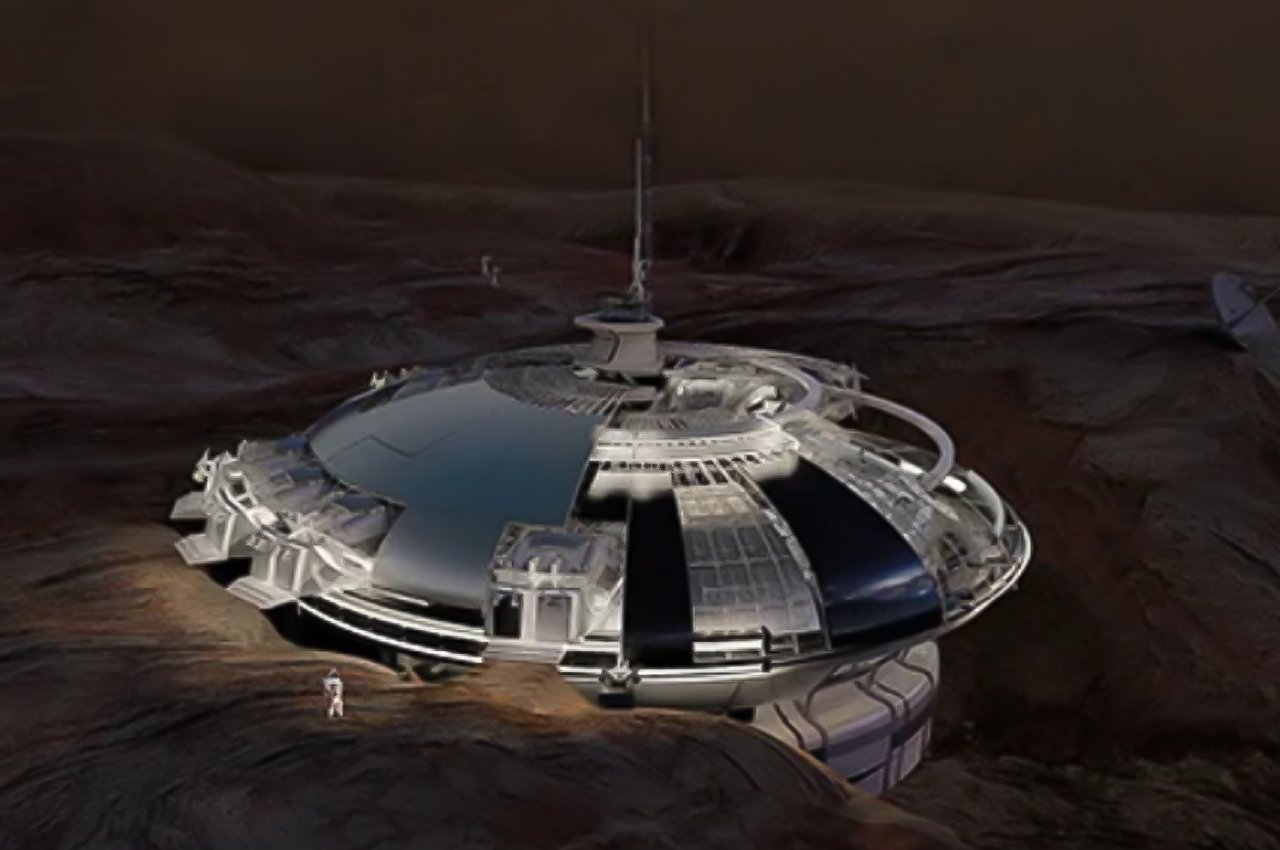The image depicts a highly detailed and realistic painting of a UFO-like structure that appears to also mimic the look of a building, possibly part of a colony on an alien planet. This circular, predominantly white structure features an antenna-like spire or smokestack rising from its top and several entryways or steps leading inside. The UFO rests on a pedestal within a barren, sandy, and hilly moonscape, set against a dark brown background that blends seamlessly with the near-dark sky. A small, white figure—perhaps a human or alien—is seen walking toward the structure, with traces of blue tinting on parts of the UFO. There might be another figure in the obscured background, suggesting a deserted or sparsely populated otherworldly environment. Despite the darkness, the scene is partially lit, highlighting the central figure and its approach to the enigmatic structure.